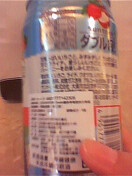In this blurred photograph, a sizable medicine or vitamin bottle is prominently featured, held securely in someone’s hand. The person's thumb is visible, indicating the bottle is quite large. The bottle's label is primarily blue, white, and orange, with a slight metallic sheen, suggesting a modern or premium design. The text on the label is indiscernible, written in a foreign script that could be Cyrillic or possibly an Asian language, making it challenging to identify the specific type of vitamins or medicine contained within. This image captures a moment of someone examining an unfamiliar health product.